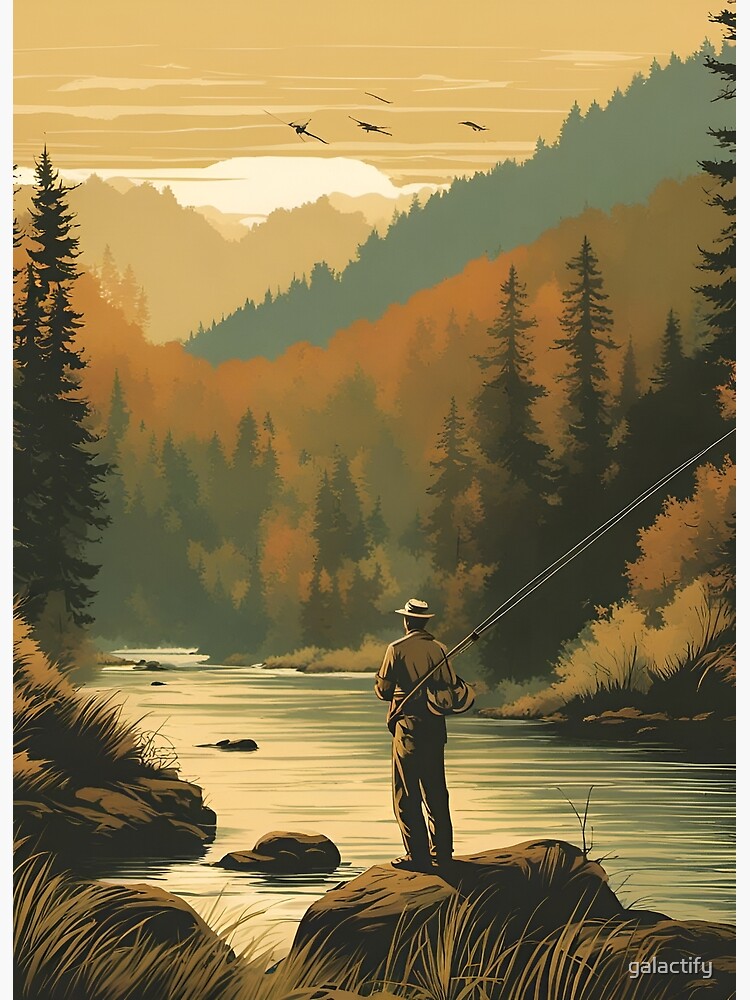In the painting, a man is depicted standing on a large brown rock at the edge of a serene river, engaged in fly fishing. Dressed in a combination of white fedora or straw hat, dark shirt, and trousers, he is holding a long fishing rod, its line casting out toward the calm waters. The water in front of him transitions from light yellow on the left to a green hue on the right, with gentle ripples where the colors blend. A light brown rock protrudes from the water near his position. In the background, layers of nature unfold: an initial line of orange and brown trees, followed by mountains blanketed in dark green-gray and gold hues, enhancing the scene's depth. The sky above is a dramatic mix of light and dark gray, interspersed with four black birds in flight. The foreground is adorned with leaves and grass, and a rocky outcrop with additional foliage lies to the right. Further to the right, a pine tree stands sentinel. The distant hills and mountains, shifting from orange-gold to brown, give the impression of a setting sun, adding to the overall tranquil yet vivid fall atmosphere. Ducks or birds are also visible flying against the sky, complementing the scene's harmonious interaction of man and nature.